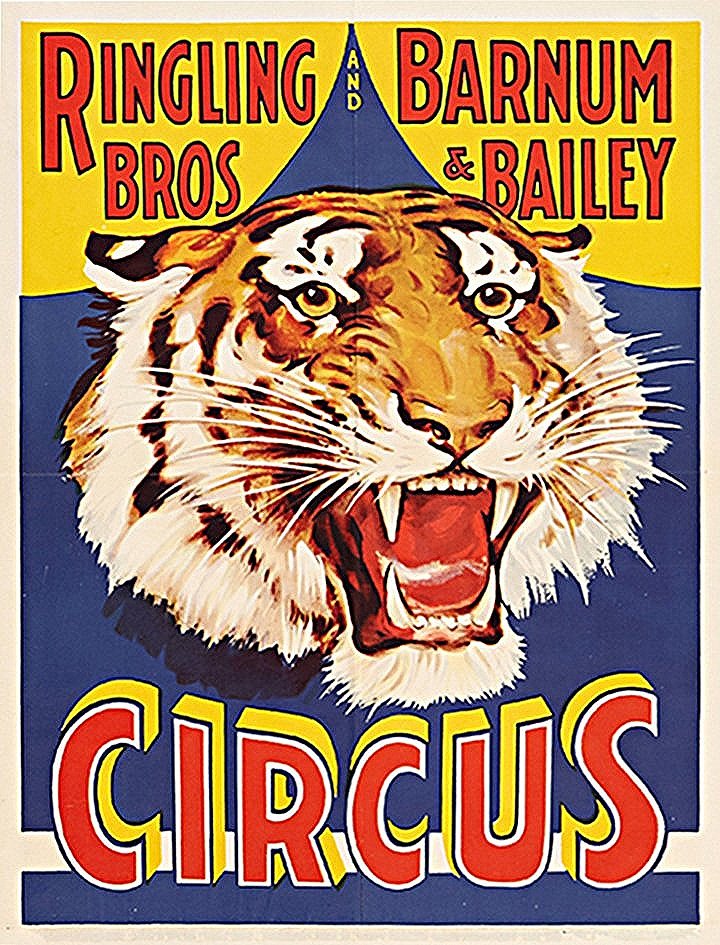This vintage-style promotional poster for the Ringling Brothers and Barnum and Bailey Circus exudes a cool, old-fashioned charm with its vivid color scheme of yellow, red, and blue. Central to the poster is a striking image of a roaring tiger with its mouth open, showcasing sharp, scissor-like teeth. The tiger's face, drawn with a cartoonish yet realistic style, features accurate detailing with orange and white fur complemented by bold black stripes. Whiskers flare out and narrowed eyes cast a glance to the side, adding to the fierce and dynamic expression. The backdrop is a deep blue circus tent set against a yellow skyline, enhancing the captivating visual impact. The poster’s bold red font is emblazoned on a yellow background, proudly proclaiming "Ringling Brothers and Barnum and Bailey Circus," with "Circus" prominently displayed in larger letters at the bottom. The overall design captures a nostalgic essence, blending vibrant colors and a striking central image to create an attention-grabbing and memorable piece.